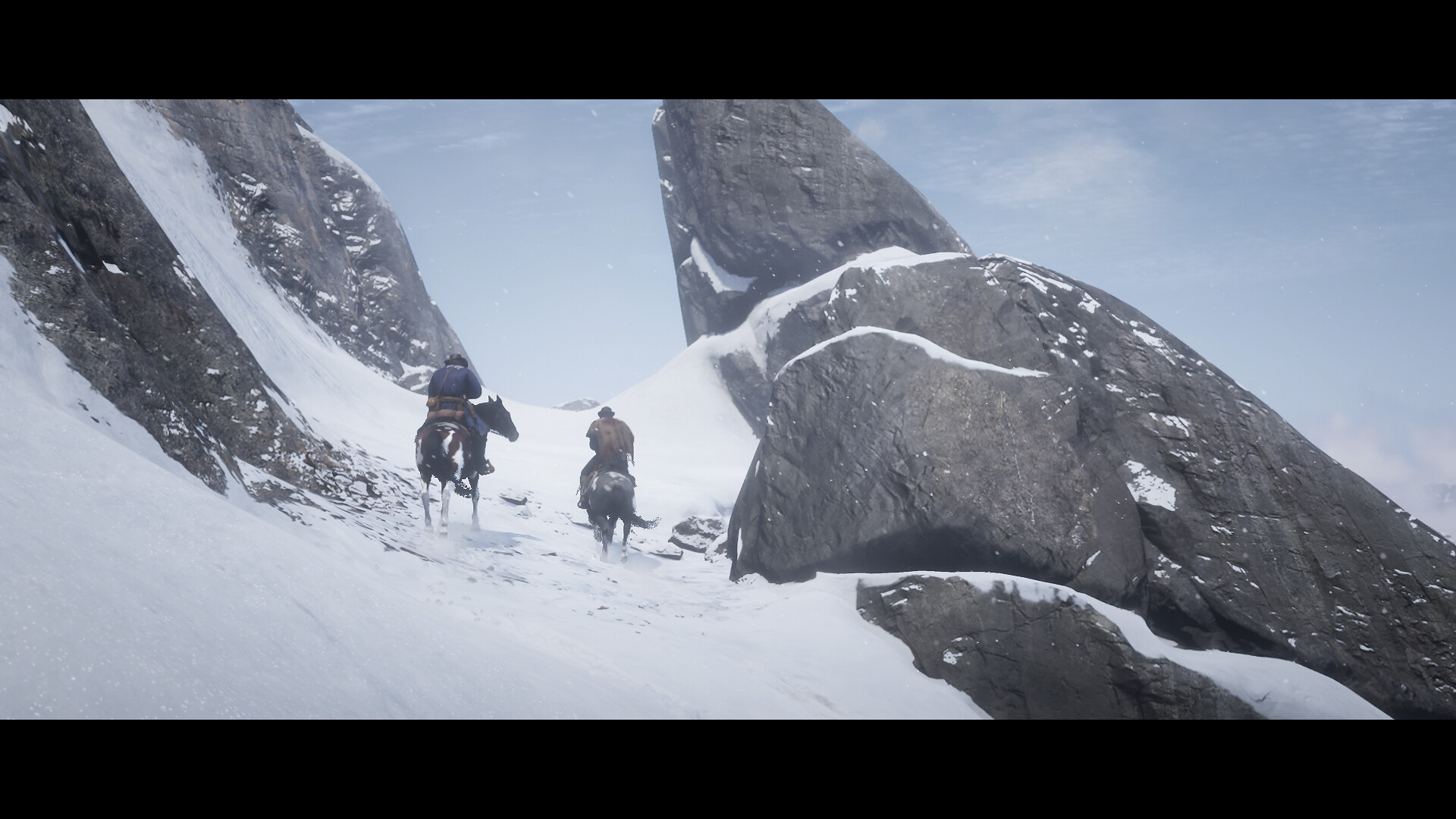This highly realistic, computer-generated image, likely from a video game cutscene or other digital media, captures an evocative scene of two men riding horseback through a rugged mountain pass. The sky above is a pale blue, providing a stark contrast to the stark, snow-covered mountains flanking the narrow passage they traverse. The tall, dark gray boulders loom imposingly on either side, creating a sense of isolation and challenging terrain. The two characters, only visible from the back, exude a palpable sense of coldness as they hunch slightly against the frigid air. They are dressed in thick, insulated coats and each wears a hat, emphasizing their preparedness for the harsh environment. Their stoic posture suggests a purposeful journey, adding a layer of narrative intrigue to the scene.